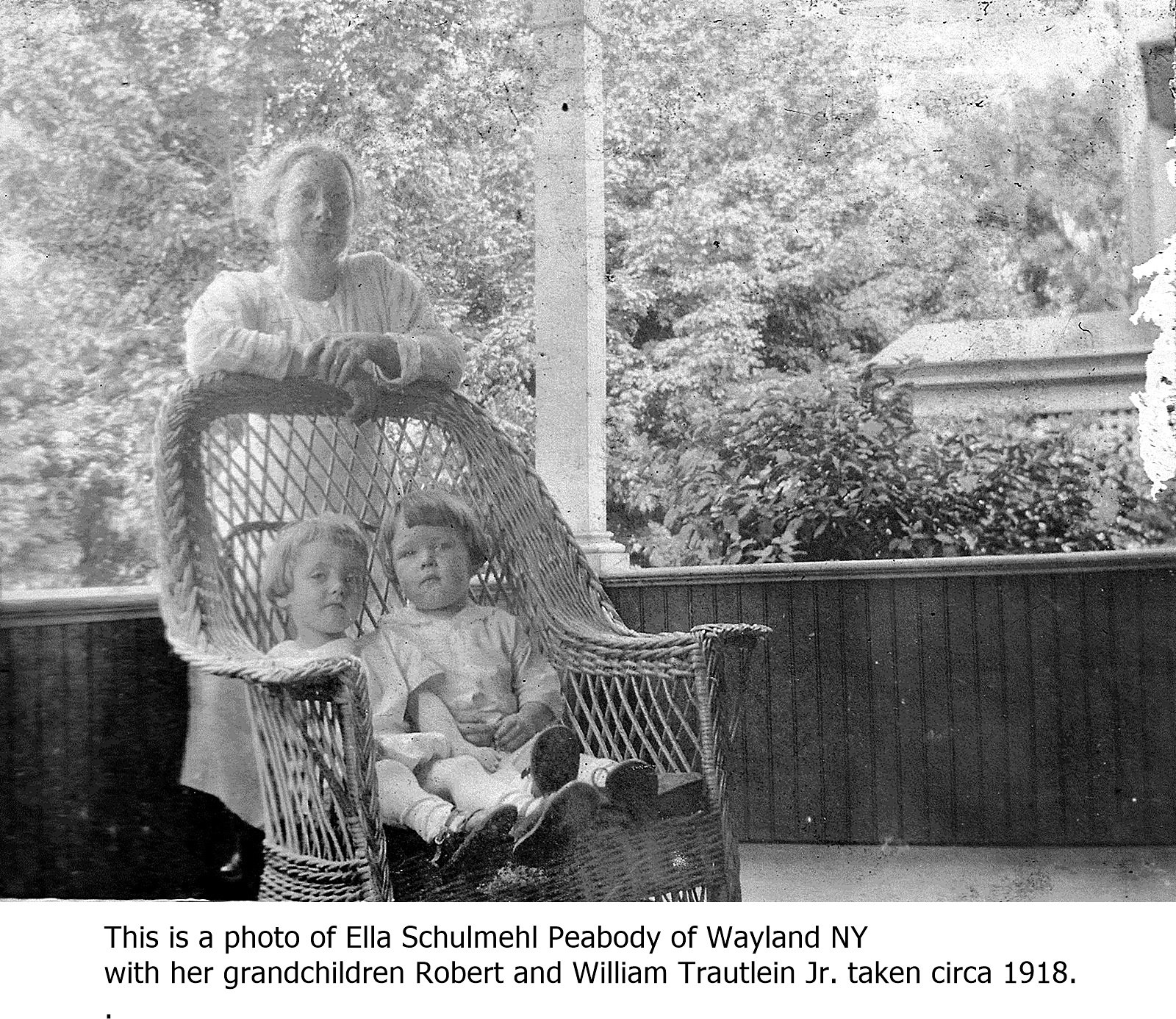In this old black and white photograph, a woman identified as Ella Shumily Peabody of Wayland, New York stands behind a large wicker chair, leaning her arms on its back. She wears a long white dress with long sleeves and has her gray hair pulled back. Her expression is neutral, with her mouth closed and her eyes difficult to discern due to the grainy quality of the image. Seated side by side in the chair are her grandchildren, Robert and William Troughton Jr., who are dressed in white dresses with dark-soled shoes that dangle just off the edge of the chair. The child on the left has light hair styled to just above the forehead and down past the ears, while the child on the right has darker hair similarly styled. The backdrop features white columns supporting a roof, with a large leafy tree and a darker bush positioned behind them, suggesting the scene is on a porch in a warm season. This photograph was taken circa 1918.